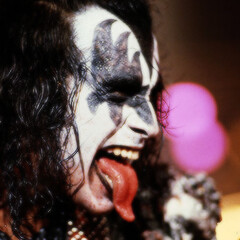An up-close profile shot of Gene Simmons from the rock band Kiss, showcasing his iconic stage look. Simmons has long, stringy black hair and is wearing his signature face paint. The upper portion of his face is painted white with intricate black star-like shapes around his eyes and a deep black triangle at the center of his forehead, obscuring his hairline. His lower jaw remains unpainted, revealing his natural skin. Simmons has his mouth wide open, sticking out his impressively long, bright red tongue, which extends down to his chin, displaying his top white teeth. The background of the image is heavily blurred, with only two large, round pink orbs visible, likely representing lights. The general backdrop features hints of tan, brown, and black colors but remains indistinct. Simmons is looking towards the far right of the image, capturing his theatrical and exaggerated stage persona.